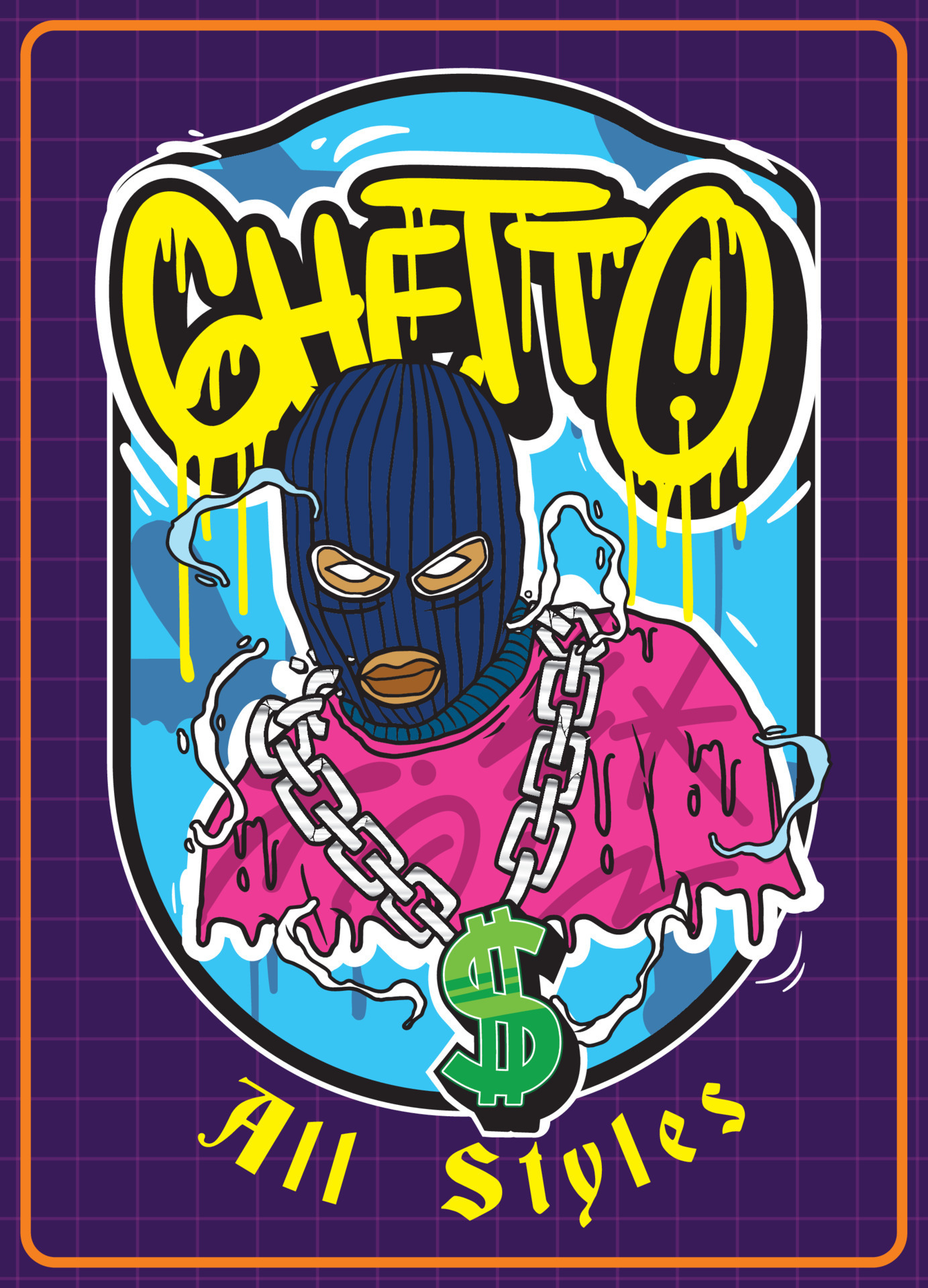The image is a detailed hand-drawn poster with a purple checkered background, featuring square grids throughout. The poster is bordered by an orange rectangle. Inside the poster, there's a blue shield-like frame with purple streaks. At the top of the shield, the word "Ghetto" is prominently written in an artistic, graffiti-style font, with an exclamation point inside the "O." Below it, there is a cartoonishly drawn Caucasian man wearing a dark purple ski mask with completely white eyes. He dons a radiant silver chain with a large green dollar sign pendant and a pink shirt adorned with darker pink designs and smoke trails around him. At the bottom of the image, the words "All Styles" are inscribed in a yellowish font.